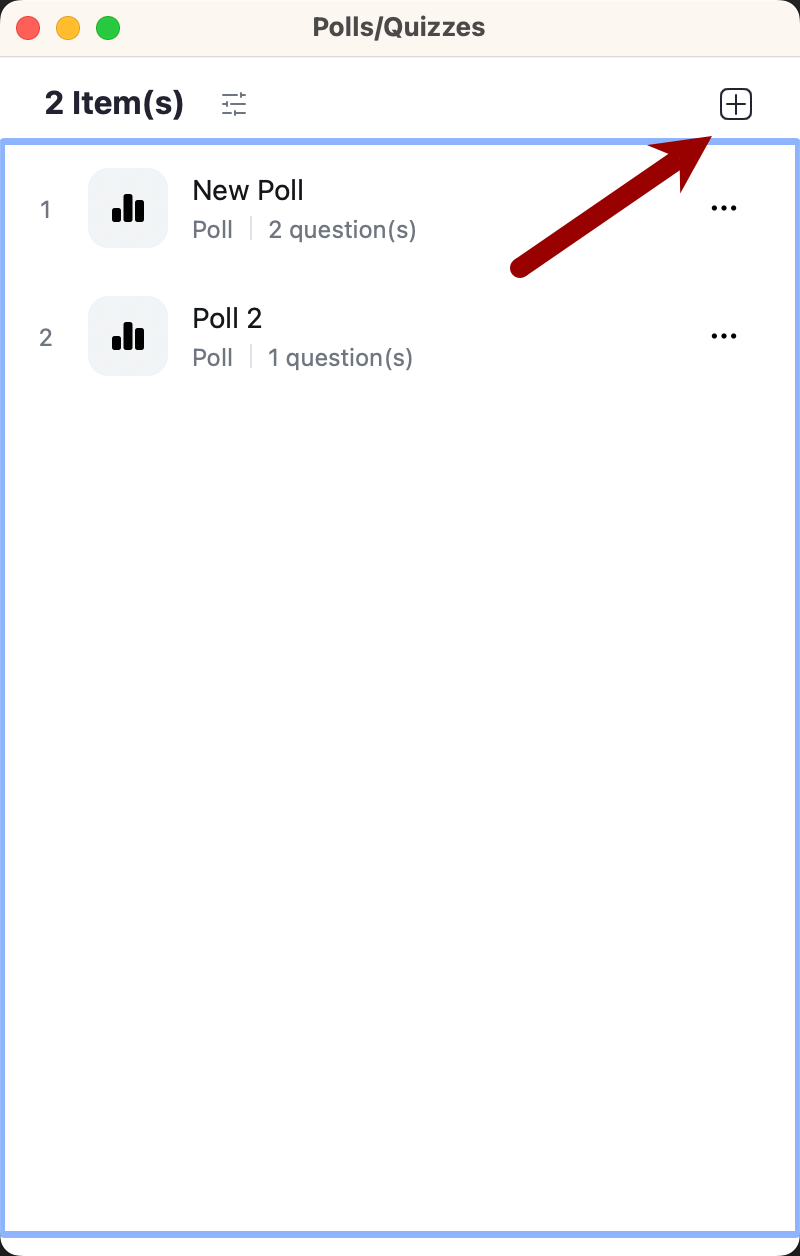This image displays a screenshot of a smartphone interface, showcasing various elements related to an app, possibly a quiz or survey application. At the top of the screen, there's a navigation bar with three colored circles: red, orange, and green. The function of these circles is unclear, but they could potentially be indicators for different statuses or actions. Immediately below this bar, the text "Pulse/Quizzes" is prominently displayed in black. Below this, there is another line of black text stating "Two items."

Further down, the screen features the "TAD" logo centered on a white background. Encasing this section is a blue rectangular outline resembling a bubble. Beneath the logo, a numbered list is visible. The first item on the list is labeled "Poll 1" and is described as a poll containing two questions. The second item is titled "Poll 2," indicating another poll but with only one question. Adjacent to these entries, a dark red arrow points towards a plus sign icon, suggesting an option to add new items or create additional content.